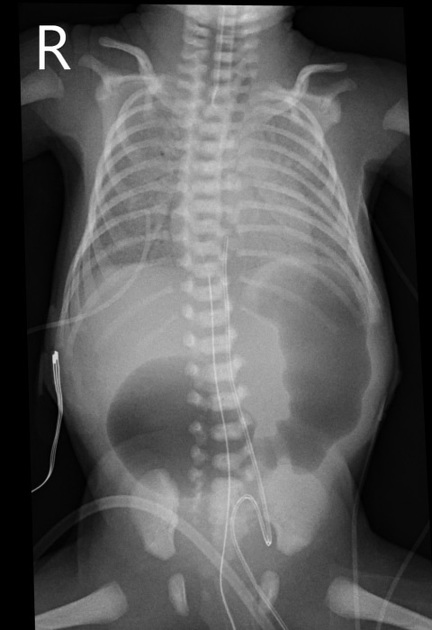This image is a detailed x-ray photograph, predominantly black with translucent white aspects that reveal various anatomical features. Central to the image is the spine, running vertically and exhibiting a slight curvature. Surrounding the spine, the ribcage is clearly visible, expanding outward with noticeable width. The image captures the skeleton from the neck down to the pelvis, where the leg bones begin but are not fully shown. The x-ray also includes the chest and back bones, emphasizing the entirety of the upper body's bone structure. In the top left corner, there is a prominent white letter "R" marking the side of the body x-rayed. The clarity of the bones contrasts sharply against the dark background, making the intricate details of the skeletal system distinctly visible.